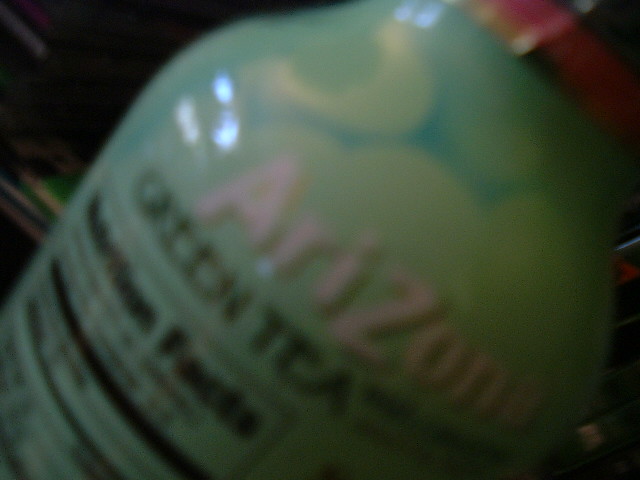This color photograph captures a close-up, out-of-focus image of the top portion of an Arizona Green Tea can. The can, with its characteristic teal color and lined with small yellow puffs, dominates the frame. Despite the blurriness, the pink Arizona lettering is discernible, positioned vertically, with "Green Tea" in black letters just below it. The image prominently features the ingredients label, although both the label and the nutritional facts are too blurry to read distinctly. The can appears to be made of laminated plastic, and the surrounding area around the can is dark, making the teal and pink colors stand out even more. The top of the can tapers slightly, hinting at a smaller opening, though specific details remain obscured due to the lack of focus.